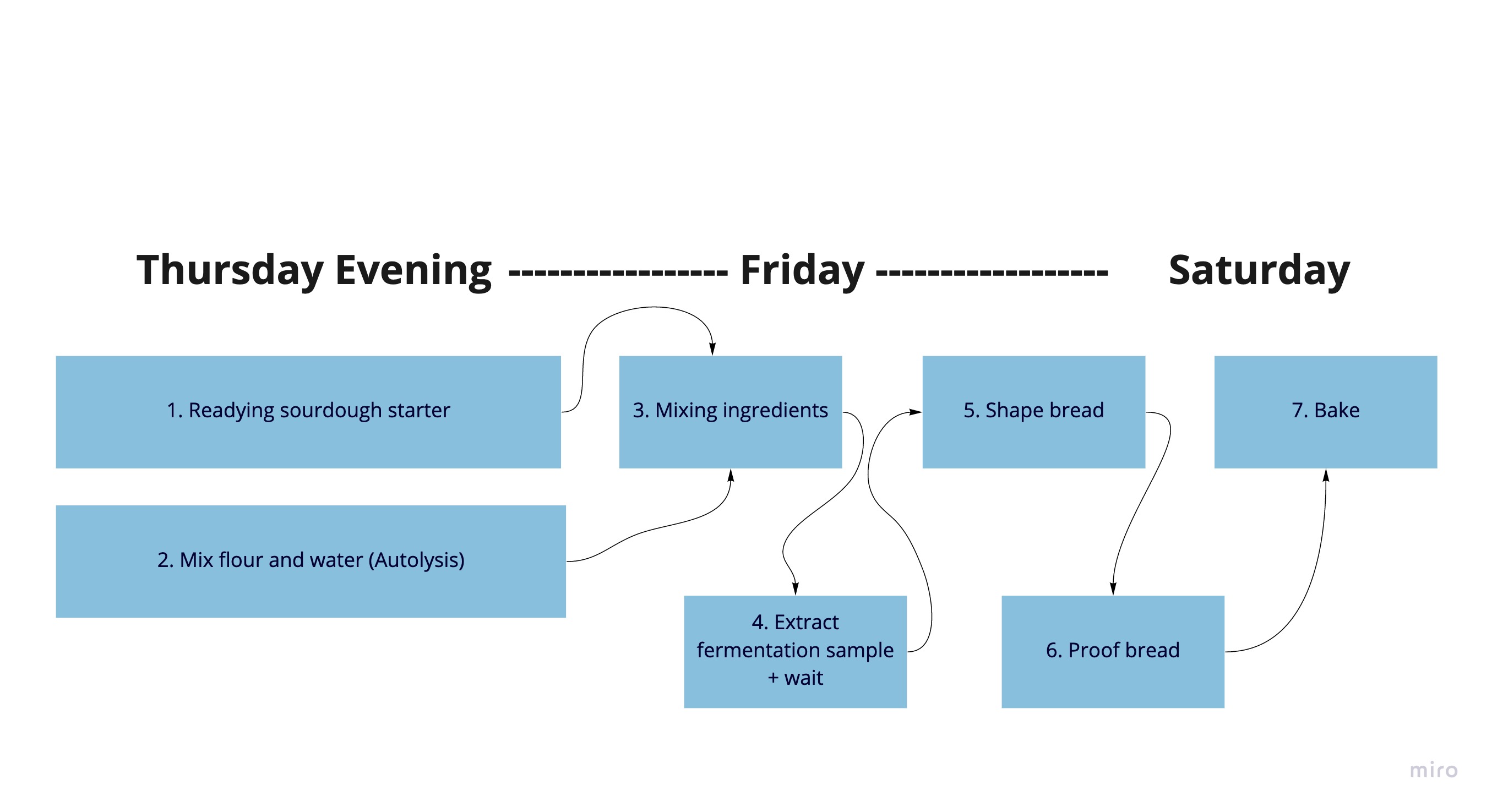This is a diagram illustrating a detailed timeline for baking bread over three days, set against a white background. At the top of the image, bold black letters label the days: "Thursday evening," followed by a dashed line leading to "Friday," with another dashed line ending at "Saturday." Below these headings, the steps are organized into blue rectangles, wider than they are tall, with each step described in blue text.

The process begins on the upper left corner under "Thursday evening" with the first rectangle labeled "1. Readying Sourdough Starter." Directly below it, the second rectangle reads "2. Mixed Flour and Water" followed by "(Autolysis)." Arrows extend from these two boxes to a third rectangle that says "3. Mixing Ingredients" which falls under Friday's heading.

Continuing on Friday, a line with an arrow connects from the third step to the fourth rectangle, which is labeled "4. Extract Fermentation Sample plus Weight." From there, another arrow leads to the fifth rectangle, stating "5. Shape Bread." Moving further along, an arrow connects to the sixth rectangle, "6. Proof Bread."

Finally, a line with an arrow points to the seventh and last rectangle under Saturday, which reads "7. Bake."

The entire diagram uses primarily black and blue colors, signifying the different steps in the bread-making process across the three days.